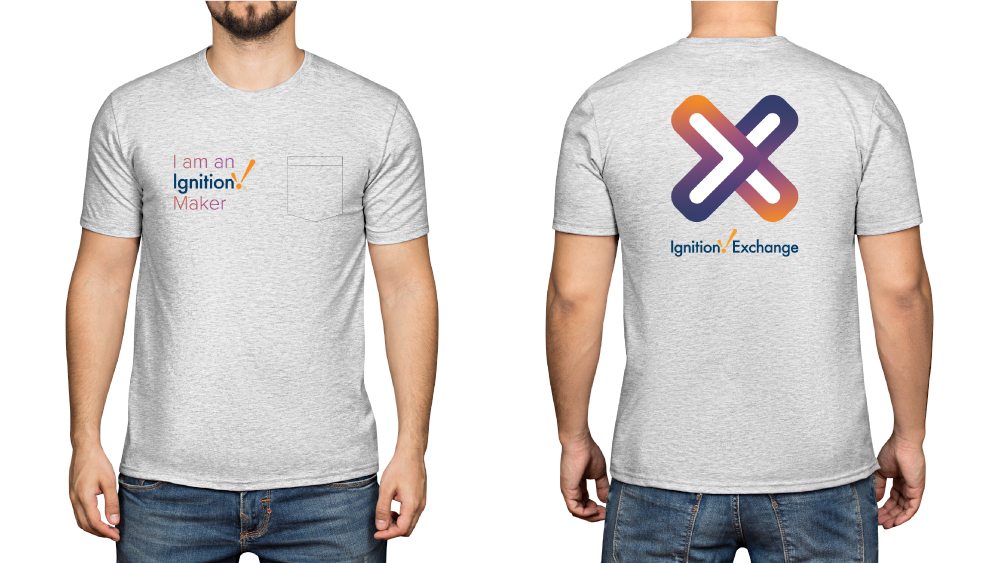The image is a detailed color photograph, possibly a computer illustration, featuring a young Caucasian man, approximately in his 30s, shown in both front and rear views. The man has a brownish goatee or short beard and is of average build. He is wearing a heathered gray t-shirt with a chest pocket. On the front, the t-shirt displays the text "I am an ignition maker" with "Ignition" written in blue and accompanied by a gold checkmark. He is also wearing normal blue jeans and stands with his arms relaxed by his sides. The back view of the t-shirt features a large X logo in violet, blue, and orange, positioned above the text "Ignition Exchange."